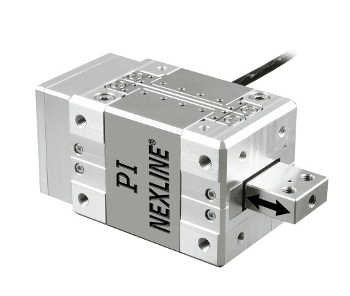The image features a machined aluminum device labeled "Pi NextLine" on one side. The device is a rectangular block with a smaller protruding section that resembles a USB port, although it is not one. This smaller section has a bidirectional arrow, suggesting it is designed to be inserted and removed, possibly indicating its function as a positional sensor or switch. The main body of the device has numerous threaded holes, likely for connecting wires and securing them with hex head screws. There is a black line or cable that extends from the upper right corner of the device, hinting at an electrical connection. The background of the image is stark white, emphasizing the silver-grey color of the machined aluminum block. There are subtle black shadings behind the device, which might be shadows or additional cables. The overall setting provides a clear view of the front, one side, and the top of the device, highlighting its utilitarian design and potential for various electrical applications.